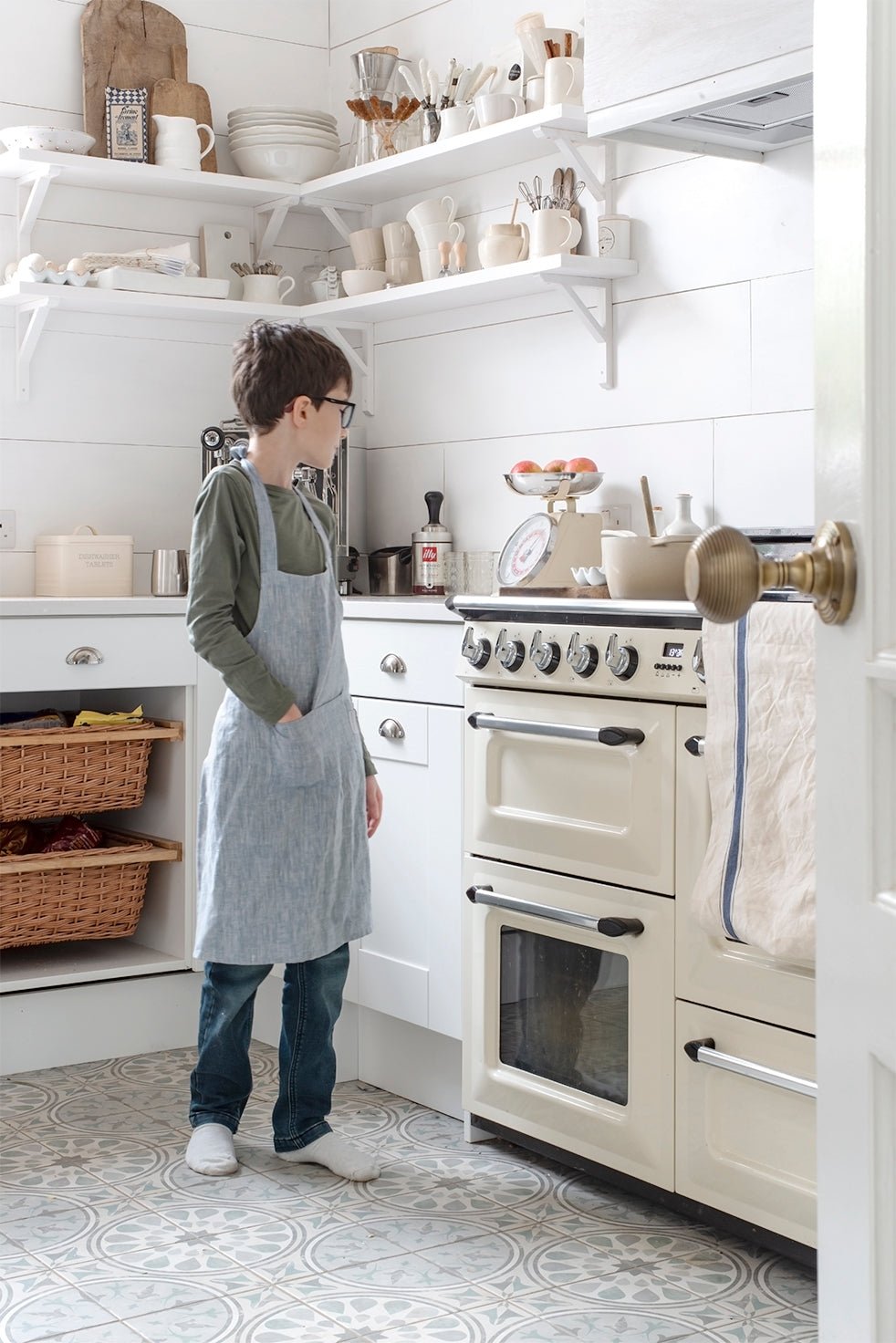In this kitchen scene, a young Caucasian boy stands in front of a cream-colored stove, focused on his cooking task. He wears a light blue apron over an olive green long-sleeved shirt, paired with blue jeans and white socks. His short black hair is slightly tousled, and he sports black-framed glasses. The kitchen is immaculate, with white walls, shelves, and cabinets, all contributing to a clean, airy feel. 

Above the boy, the white shelving holds an array of mugs filled with utensils, plates, bowls, and various kitchen tools. Flanking the stove, wicker baskets are tucked away in a cupboard, hinting at well-organized storage. On the counter next to him, a scale holds several apples, and a container with a spoon sticking out suggests recent use in his cooking endeavors. The floor beneath him is tiled in a pattern of different shades of gray and white, complementing the kitchen's predominantly white theme. To the right, a door with a silver handle peeks into the scene, possibly leading to another room. The boy's right hand casually rests in his apron pocket as he stands immersed in his culinary activity.